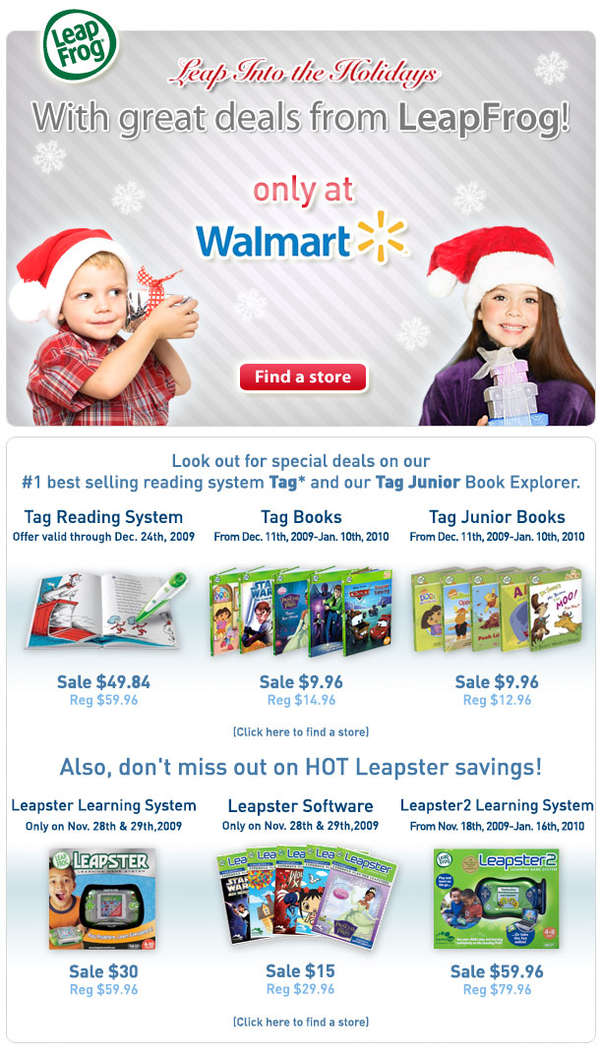"Leap into the holidays with fantastic deals from LeapFrog! Only at Walmart, find a store near you to take advantage of special offers on our top-rated reading system. Featured in the ad are various product listings, including popular children’s books at the top and innovative reading devices at the bottom. Don't miss out on exclusive savings on our number one best-selling educational tools designed to make learning fun for kids!"